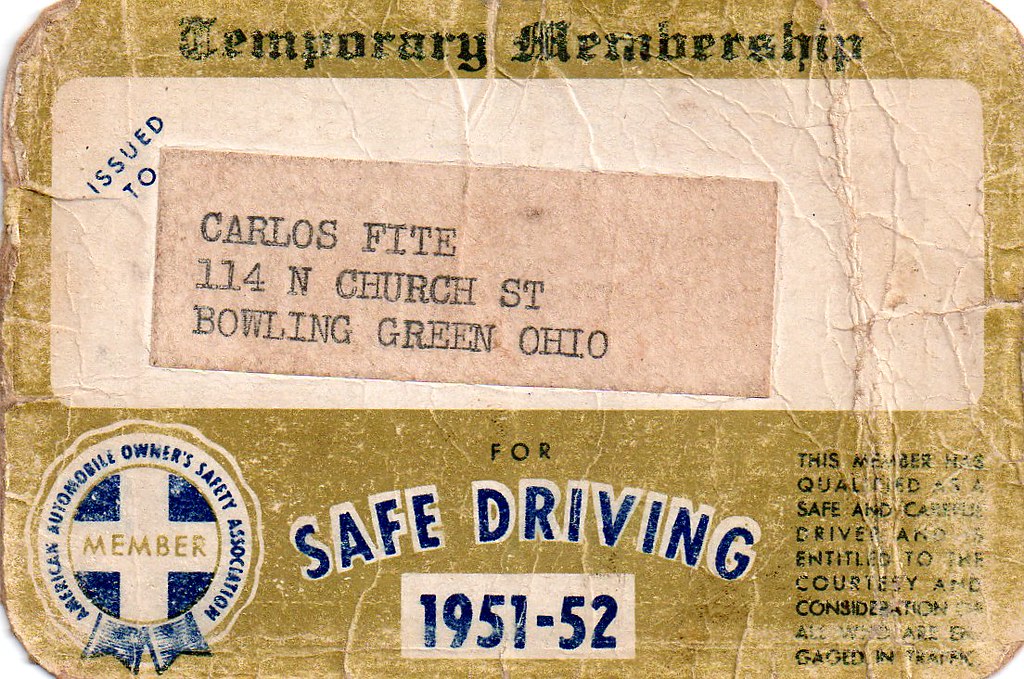The image appears to be a Xerox copy of an old, tattered temporary membership card issued for safe driving, dating from 1951-1952. The card is primarily gold with a faded greenish-yellow tint and features black text at the top that reads "Temporary Membership" in an old-timey font. Below this, a beige sticker bears the text "Issued to Carlos Fite, 114 North Church Street, Bowling Green, Ohio." The center of the card displays blue text that states "Safe Driving, 1951-52," accompanied by an emblem labeled "Member, South America Automotive Owner Safety Association." There is also a nearly illegible text indicating that the holder has qualified as a safe and cautious driver deserving of courtesy and consideration. The card appears to be a thin piece of cardboard, indicative of its age and likely professional photocopy reproduction.